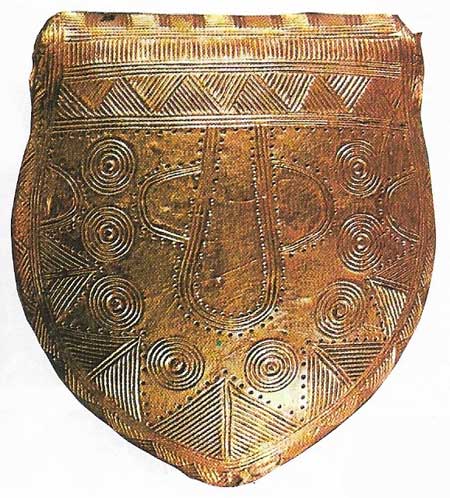The image showcases a remarkably preserved ancient bronze shield featuring a traditional design characterized by a flat top that transitions into rounded sides tapering to a point. This shield is intricately engraved, displaying an array of geometric patterns, including numerous triangles filled with cross-hatched lines and concentric circles. A standout feature is a downward loop in the middle, backed by an oval pattern, and bordered with delicate pinprint designs. The surface also exhibits little dots, swirls, and beige stripes near the top, all contributing to a complex and visually rich aesthetic. Despite its age, the shield retains a stunning bronze hue, indicative of its significant historical value. The background is white, which contrasts sharply with the artifact, allowing the detailed engravings and the bronze color to stand out prominently.